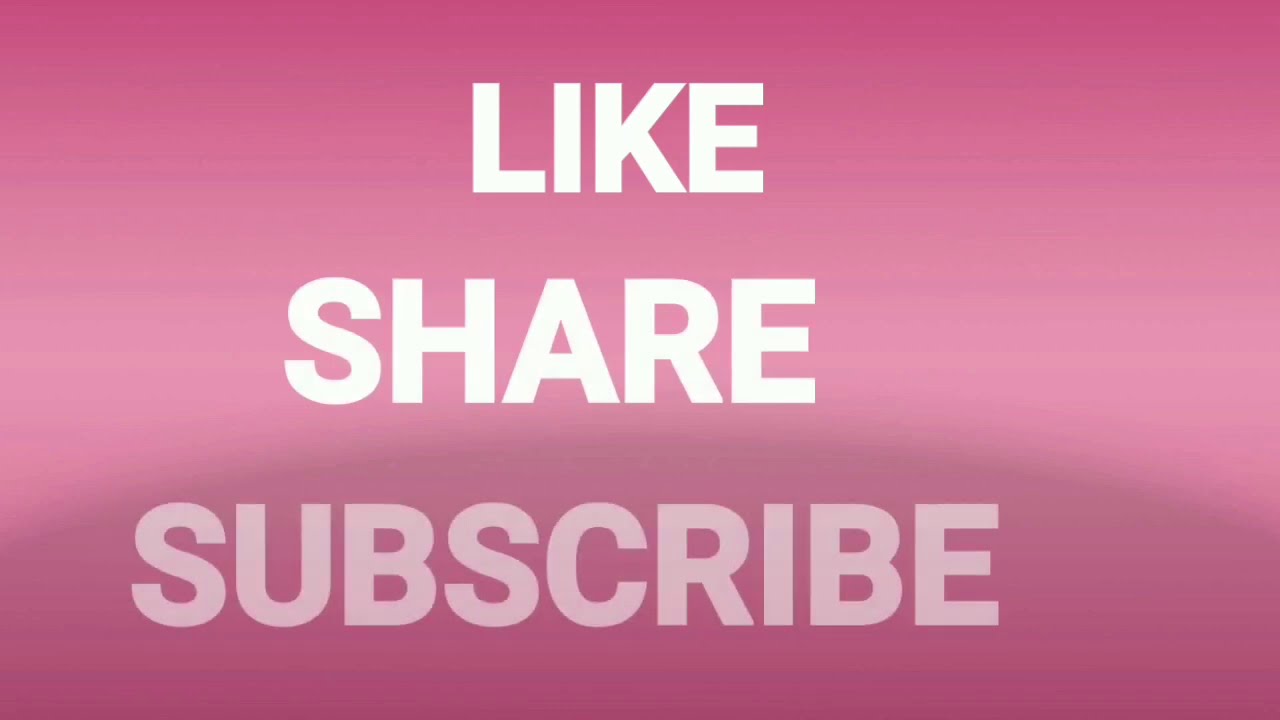The image features a horizontal rectangular layout with a captivating pink gradient background that seamlessly transitions from darker pink at the top and bottom to a lighter, almost whitish hue in the center. Faint, horizontal lines in purplish tones can be observed running through the gradient, possibly due to compression artifacts. At the center of the image but slightly skewed to the left, there are three prominent, capitalized words arranged vertically: "LIKE" at the top, followed by "SHARE" in the middle, both in bold white text, and "SUBSCRIBE" at the bottom in a subtle light pink color. This aesthetically pleasing design, with its harmonious blend of pink and white hues, appears to serve as a call-to-action notice, perhaps encouraging viewers to engage with some form of online service or content, although specific details about the service are not provided.